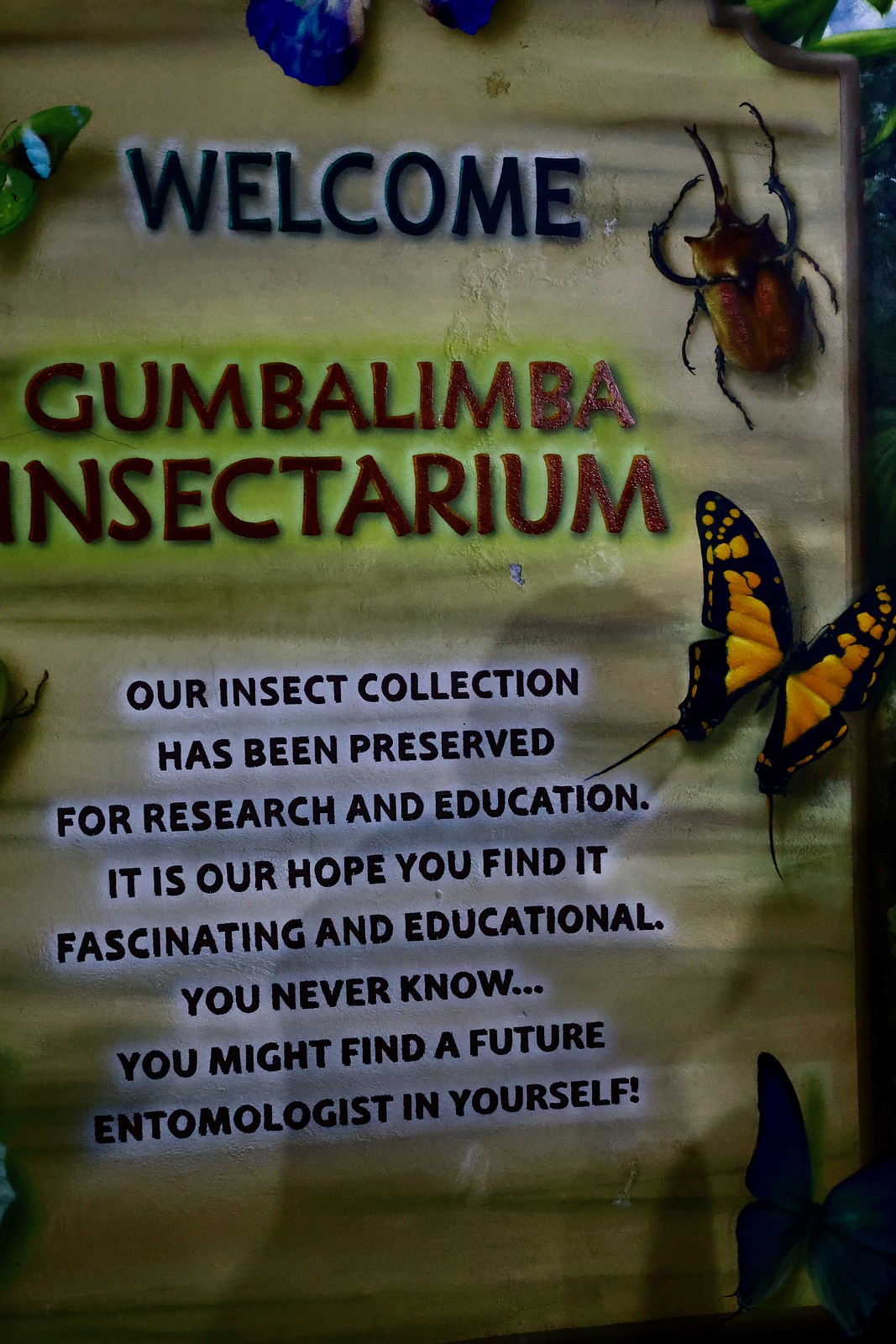The image depicts a vertically-oriented wooden sign situated in front of a building. The sign prominently features text and various artistically drawn and painted insects. At the top, against a green background, the word "Welcome" is written in blue. Below, "Gumbalimba Insectarium" is inscribed in brown. Directly beneath this, in black text, it reads: "Our insect collection has been preserved for research and education. It is our hope you’ll find it fascinating and educational. You never know when you might find a future entomologist in yourself."

The top right corner of the sign showcases a brown beetle, while the middle section is adorned with a yellow and black butterfly. Additionally, a blue and white butterfly is located towards the center-right, and a green and blue moth accompanies it nearby. In the bottom right corner, a dark, almost black butterfly is depicted. Lesser visible bugs can also be seen along the top and sides, contributing to the sign's appeal. The background transitions from light green at the center to a lighter brown shade at the top. The intricate details and text work together to encourage viewers to explore the insect collection and spark interest in entomology.